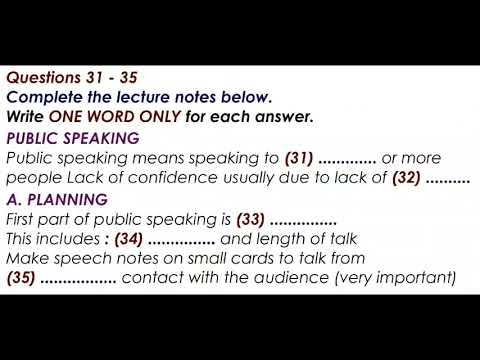The image displays a square perspective slide with thick black letterbox bars at the top and bottom, framing a solid white center filled with instructional text. The slide features various lines of text categorizing and instructing on a lecture completion exercise. 

At the top, in bold, italics, and red font, the slide states: "Questions 31-35". Below, in purple, it instructs: "Complete the lecture notes below". Following that, a black text command reads: "Write one word only for each answer". 

The main content begins with a purple heading: "Public Speaking", followed by a series of lines formatted to guide note completion:
- "Public speaking means speaking to (31) or more people."
- "Lack of confidence usually due to lack of (32)."
- "A planning."
- "First part of public speaking is (33)."
- "This includes (34) and length of talk."
- "Make speech notes on small cards to talk from (35)."

Final remarks include: "Contact with the audience (very important)" appended in parentheses. The text throughout varies in color from red to purple to black, with key headings typically in purple and additional details in regular black font.